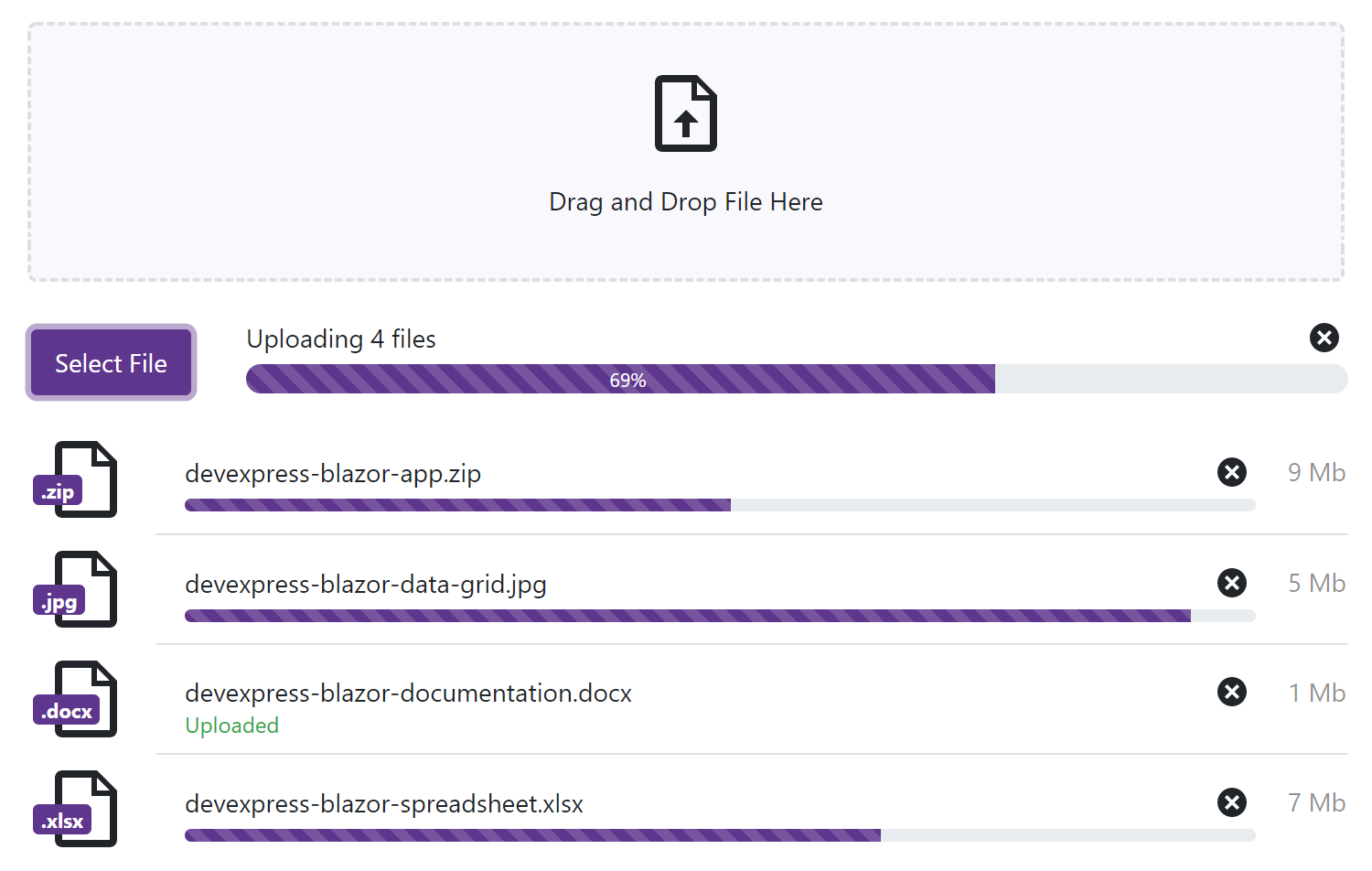This image is a screenshot of what appears to be a web application featuring a purple, black, and white color scheme. The top quarter of the image is a blank gray space, highlighted by an icon of a page with a dog-eared corner in the upper right, and an upward-pointing arrow on the page. Below this icon, the text "Drag-and-drop file here" indicates where users can drag their documents or zip files for upload.

Beneath this instruction is a purple button with white text that reads "Select File." A status bar below the button displays the ongoing upload progress, currently at 69%, with the gray bar now 69% filled with purple. 

Further down, the documents being uploaded are listed, which include:
1. A 9 megabyte zip file
2. A 5 megabyte JPEG
3. A 1 megabyte document
4. A 7 megabyte spreadsheet